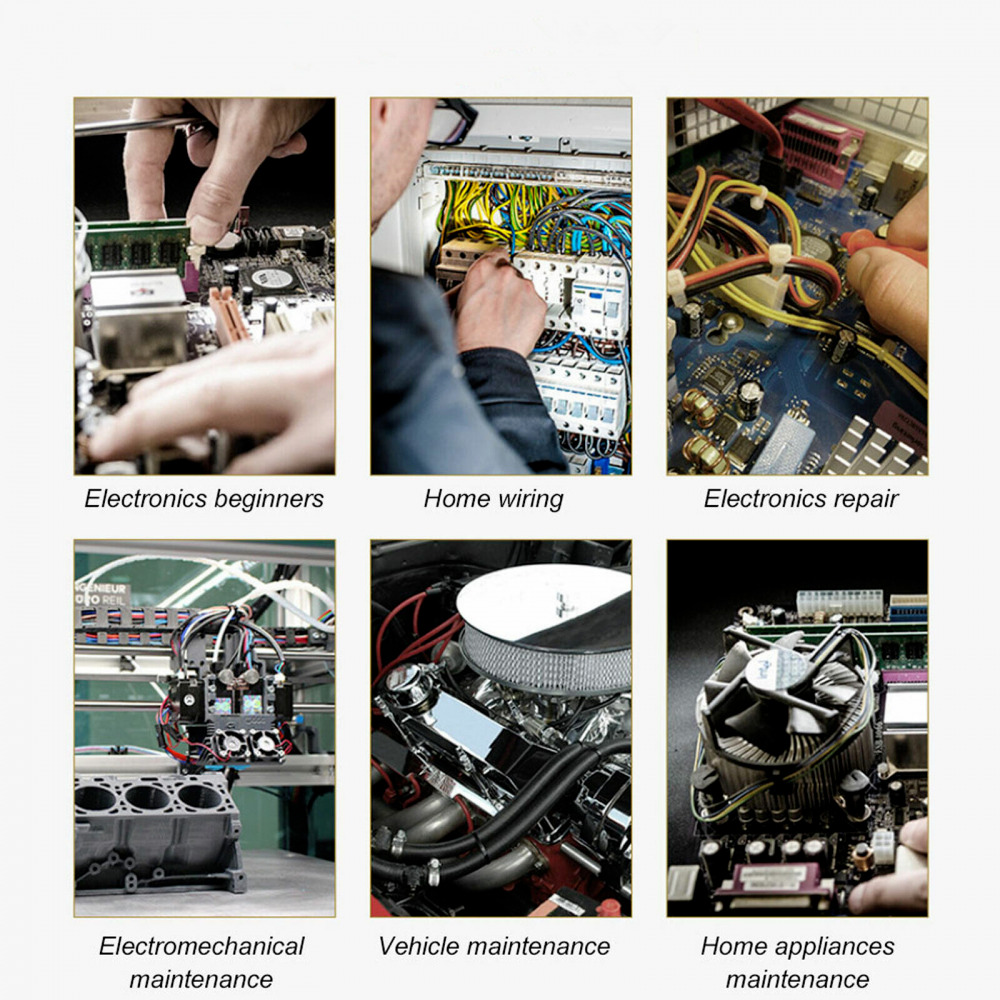This image is divided into six panels arranged in two rows of three. Each panel showcases a different aspect of electronics and maintenance work, accompanied by descriptive text below. The top left panel, labeled "Electronics Beginners," depicts a pair of hands manipulating a motherboard, suggesting someone new to electronics. The middle panel on the top row, labeled "Home Wiring," shows a man, identifiable by his shoulder and glasses, fixing a complex network of wires. The top right panel, labeled "Electronics Repair," features a hand using a tool on multicolored wires connected to a blue motherboard, indicating a repair process. The bottom left panel, labeled "Electromechanical Maintenance," displays a 3D printer entangled with various wires. The middle bottom panel, labeled "Vehicle Maintenance," is not described in detail but likely pertains to automotive repairs. The bottom right panel, labeled "Home Appliances Maintenance," shows a part of a computer's internal fan array. Across these images, technical components like circuits, wires, and metal objects are prominent, underscoring the theme of electronic and mechanical maintenance. Human hands are visible in four of the panels, adding a layer of practicality and human interaction to the technical scenes.